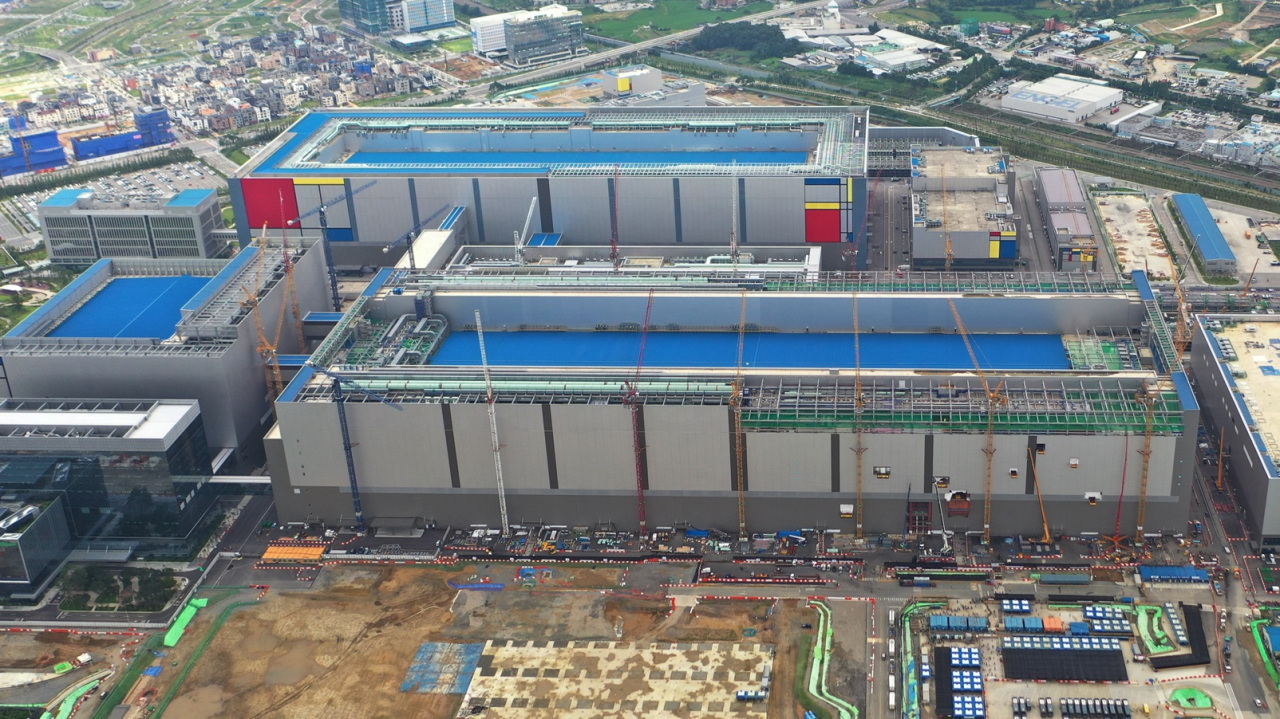The image is a detailed aerial shot, likely captured from a helicopter or drone, showcasing a large industrial complex amidst a vibrant environment. Central to the image are three sizable buildings under construction, arranged in a way that forms a connected facility with potential bridges and walkways linking them. The largest building stretches horizontally from left to right, with cranes and latticework signaling ongoing construction work around it. Adjacent to this, a smaller rectangular building sits below to the left, and another rectangular structure is positioned behind it, each seemingly covered with blue tarps. 

The bottom fourth of the image features a brown, dirt-filled construction area, while the upper portions display a mix of greenery and urban elements. The top right shows distant buildings, possibly resembling an airport, surrounded by patches of grass and trees. To the top left, more buildings and possibly houses are visible, suggesting a suburban or residential area nearby. The image, devoid of any text, is bathed in natural daylight, ensuring a bright and clear view that highlights the diverse colors present—blue, gray, white, brown, green, red, and yellow. On the periphery, streets lined with tiny cars indicate the expansive size of the construction site, which seems to occupy several city blocks in this bustling, brightly-lit outdoor setting.